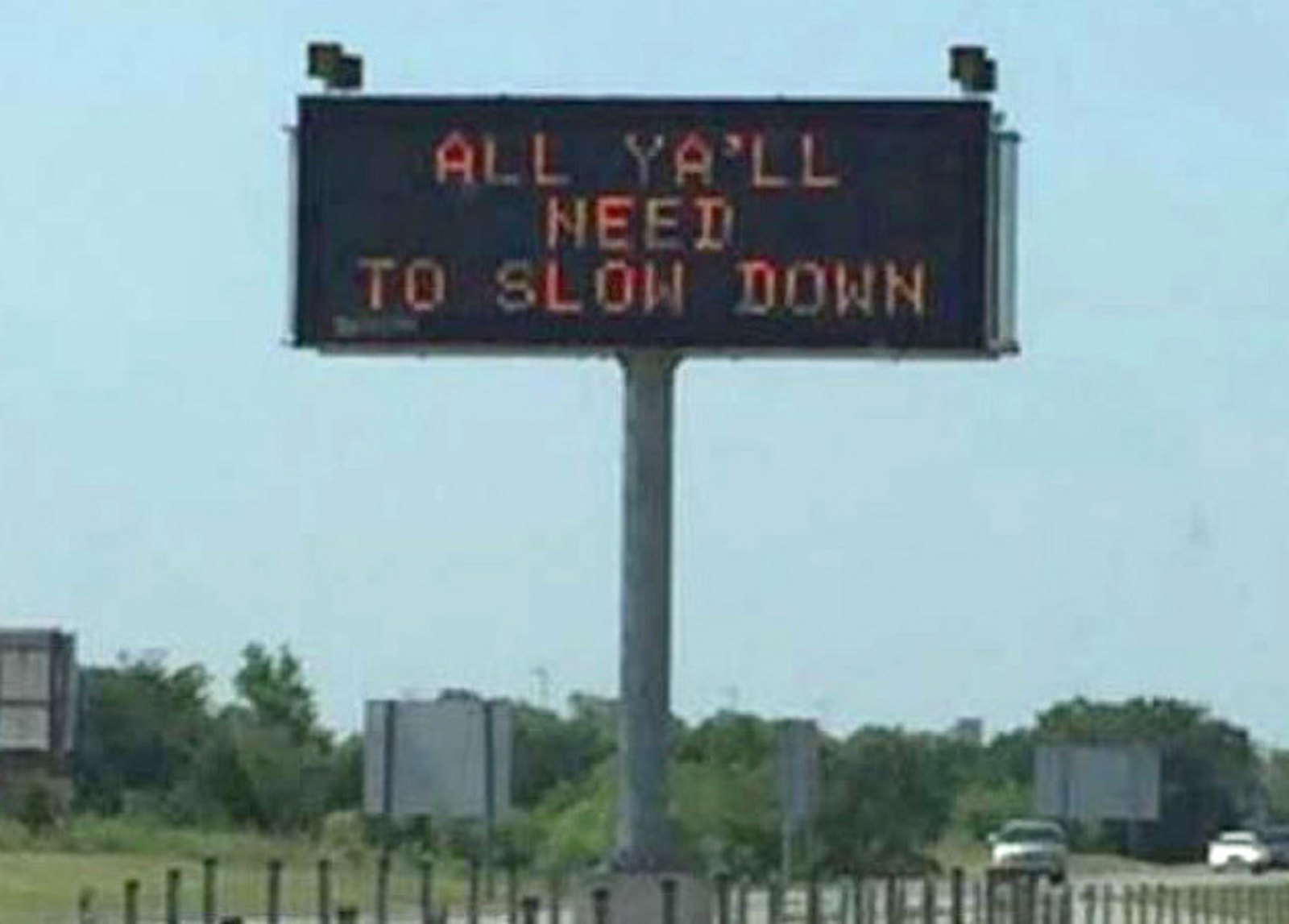This image captures a brightly illuminated electronic street sign situated along a southern interstate, positioned to deliver changeable messages to passing traffic. The current message humorously advises, "All y'all need to slow down." The vantage point of the shot is from the right-hand lane, providing a clear view of oncoming vehicles in the distance. The scene is bathed in the warmth of a beautiful southern day, characterized by a bright blue sky and lush, green trees in full bloom that frame the background. Additional billboards are partially visible, their reverse sides subtly lining the road, but the electronic sign at the center draws all the attention with its timely message.